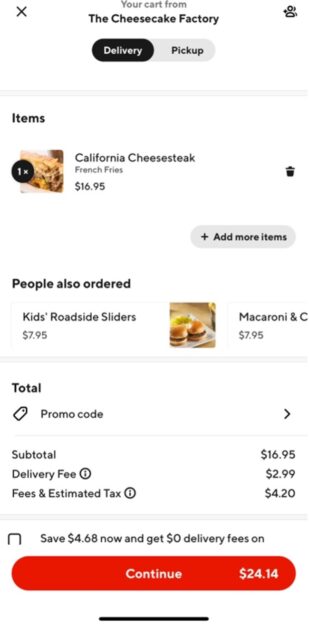Screenshot of the Cheesecake Factory's online ordering page:

At the top of the webpage, there's a title indicating "Your Cart from The Cheesecake Factory." The options for "Delivery" are highlighted in black, while "Pickup" is shaded in gray, and an 'X' icon is located on the left side for closing the cart. On the right side, there is an image that appears to show people.

The next section is labeled "Items," showing a California Cheesecake with a quantity of one, priced at $16.95. On the right side of this item, there's a trash icon for removing it from the cart. Below that, there's a gray circular button labeled "Plus add more items."

Additionally, there is a suggestion section titled "People also ordered," which includes "Kids Roadside Sliders" priced at $7.95 and "Macaroni and Cheese" also at $7.95. A partially visible picture of the sliders is shown, while the image for the macaroni and cheese is cut off.

The cost breakdown is as follows: the subtotal of $16.95, delivery fee of $2.99, and estimated fees and tax totaling $4.20. There is an information icon represented by a circle with an 'i' inside it next to the fees and tax section for additional details.

A promotional box offers savings of $4.68 and the option for zero delivery fees, with a red "Continue" button next to it. The total cost is displayed as $24.14 to the right of this promotional box.

At the bottom of the page, a black bar spans near the entire width of the website.